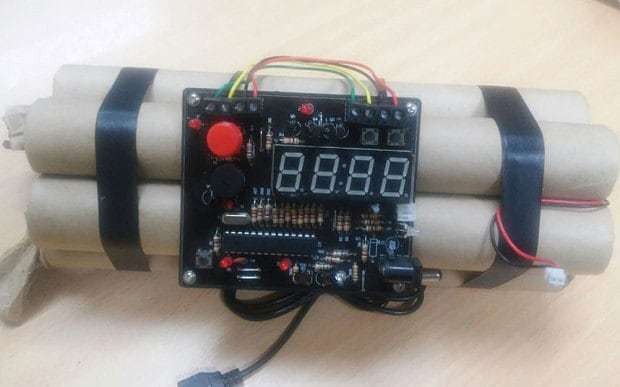The image depicts a central object that occupies around 80% of the frame, lying horizontally on a wooden surface that could be either a table or wood flooring. The object resembles a makeshift time bomb, composed of at least four brown, tube-like components that resemble sticks of dynamite, held together by black bands at either end. Attached to the middle of these tubes is an electronic circuit board with an LED display, currently displaying "8888," surrounded by multicolored resistors and other electronic components. Prominently featured on the circuit board are a big red button located at the upper left-hand corner and an array of multicolored wires (red, black, yellow, and green) extending from the top. A USB cable extends from the bottom of the circuit board. The overall color scheme of the image includes shades of brown, black, red, green, and yellow, set against a white background. The bomb is slightly slanted but mostly centered within the image, and its setup suggests it could be within someone's house or a building where it was assembled.